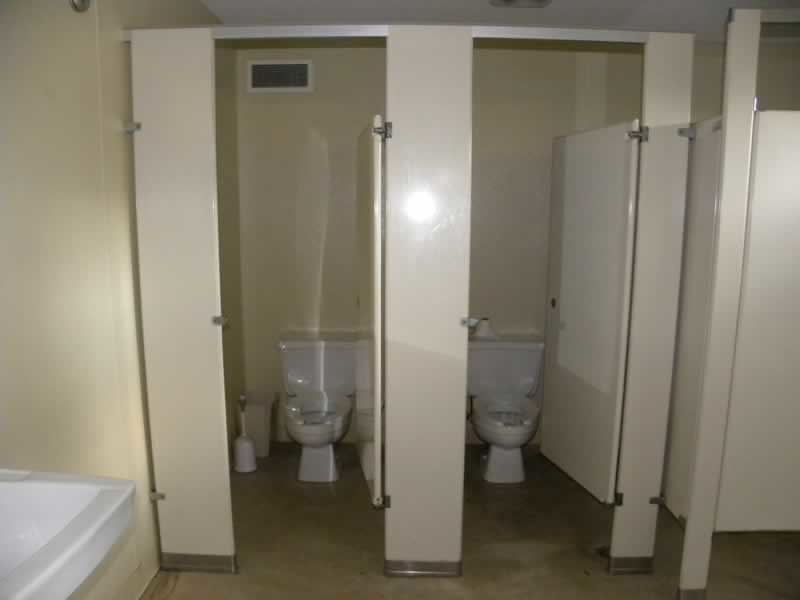This photograph captures a dimly lit, warm-toned bathroom with three stalls. The overall color palette is a uniform beige on the stalls, walls, and floor, suggesting an older, well-used facility, reminiscent of a hospital. The focus lies on two stalls with open doors, revealing white porcelain toilets, each with an open bowl. Above one stall is a white vent with a black interior, and adjacent to another stall, a white sink juts into the frame from the bottom left corner. The white elements within the bathroom contrast with the beige surroundings. Details include a plunger or cleaning brush in a container next to one toilet, and a tissue roll on the toilet in another stall. One stall door remains closed, and hinting at additional fixtures, a white object, possibly a tub, is partially visible at the photo's edge. The light reflects gently off the surfaces, adding a subtle glimmer to the scene.